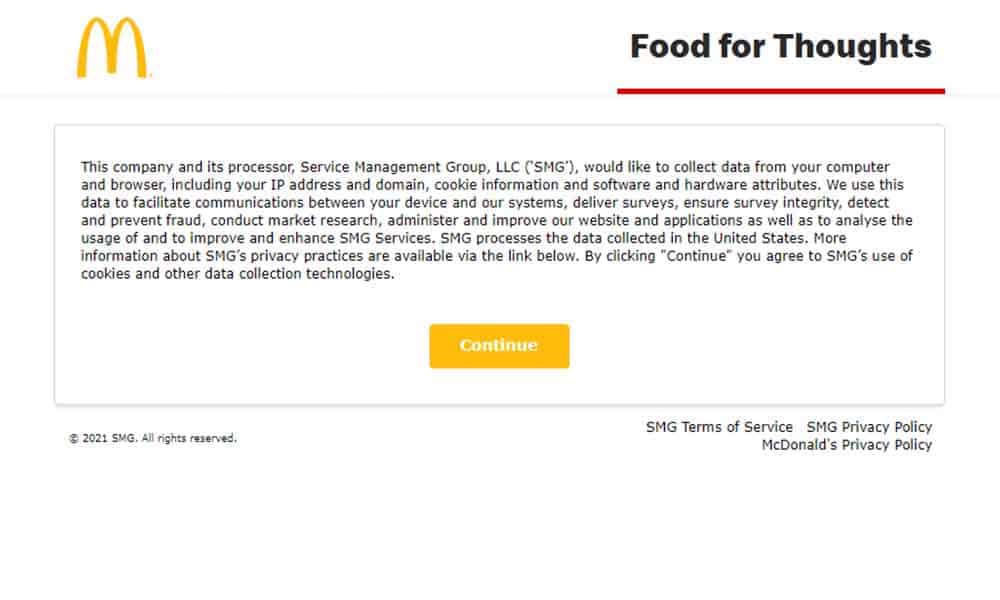This image appears to be a section of a McDonald's website. In the top left corner, there is the iconic yellow "M" logo of McDonald's. On the top right, the phrase "Food for Thought" is displayed in dark black text with a red bar beneath it. Below this header, a large rectangular box contains detailed information.

At the very bottom of the image, in a smaller section, it states "Copyright 2021 SMG. All rights reserved." On the right side of this section, there are links labeled "SMG Terms of Service," "SMG Privacy Policy," and "McDonald's Privacy Policy."

Inside the larger rectangular box, a comprehensive paragraph details SMG’s data processing practices. It explains that data is collected to facilitate communications between user devices and company systems, deliver surveys, ensure survey integrity, detect and prevent fraud, conduct market research, and improve their website and applications. This data is processed in the United States. For more information on SMG's privacy practices, there is a link provided below the text. At the bottom of this box, there is an orange rectangular button labeled "Continue."